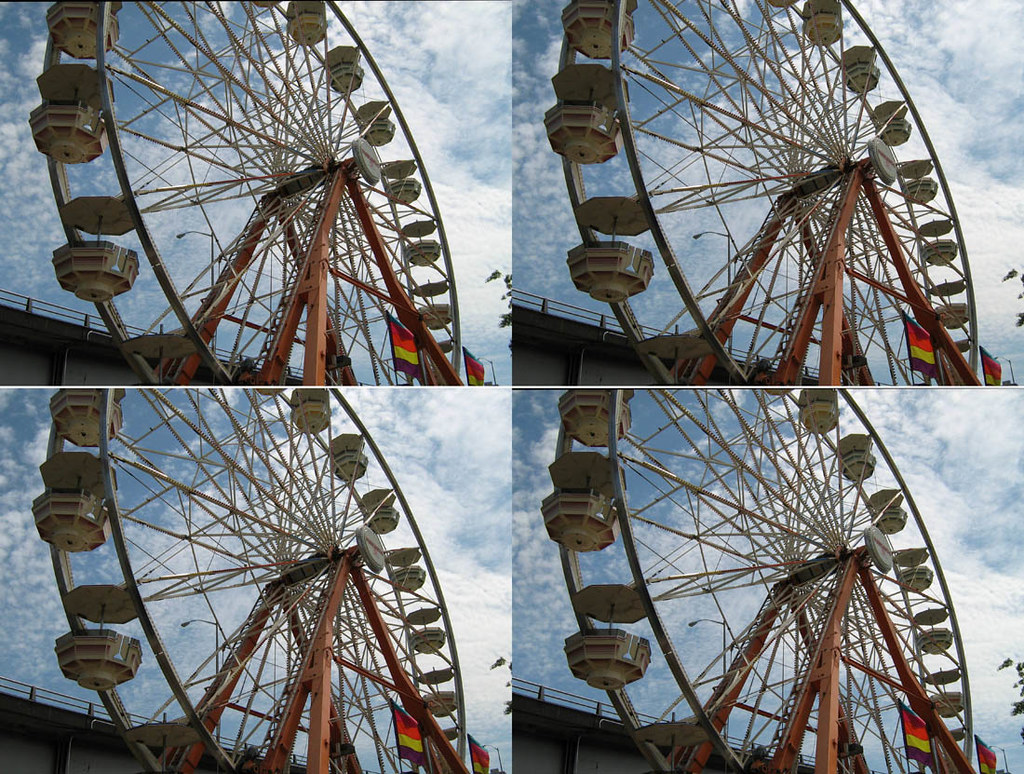The image is a composite of four photographs arranged in a two-by-two grid, each depicting an old-timey Ferris wheel from an upward angle, against a backdrop of blue sky with white clouds. All four photographs appear identical, as if taken from the same angle and under the same lighting conditions, effectively creating a seamless montage. The Ferris wheel features large metal struts in a light burnt orange color, extending at 45-degree angles toward the center. It has gondola-style cars that are open, with basket-like seats at the bottom and vertical rods supporting fixed, open umbrellas above. Visible in the back left corner behind the Ferris wheel is a bridge with a horizontally running side railing. A rainbow-colored flag with green, red, yellow, and purple segments can be seen in the bottom right corner of each photograph. The absence of passengers and the tilted upward perspective offer a clear, unobstructed view of this vintage amusement ride.